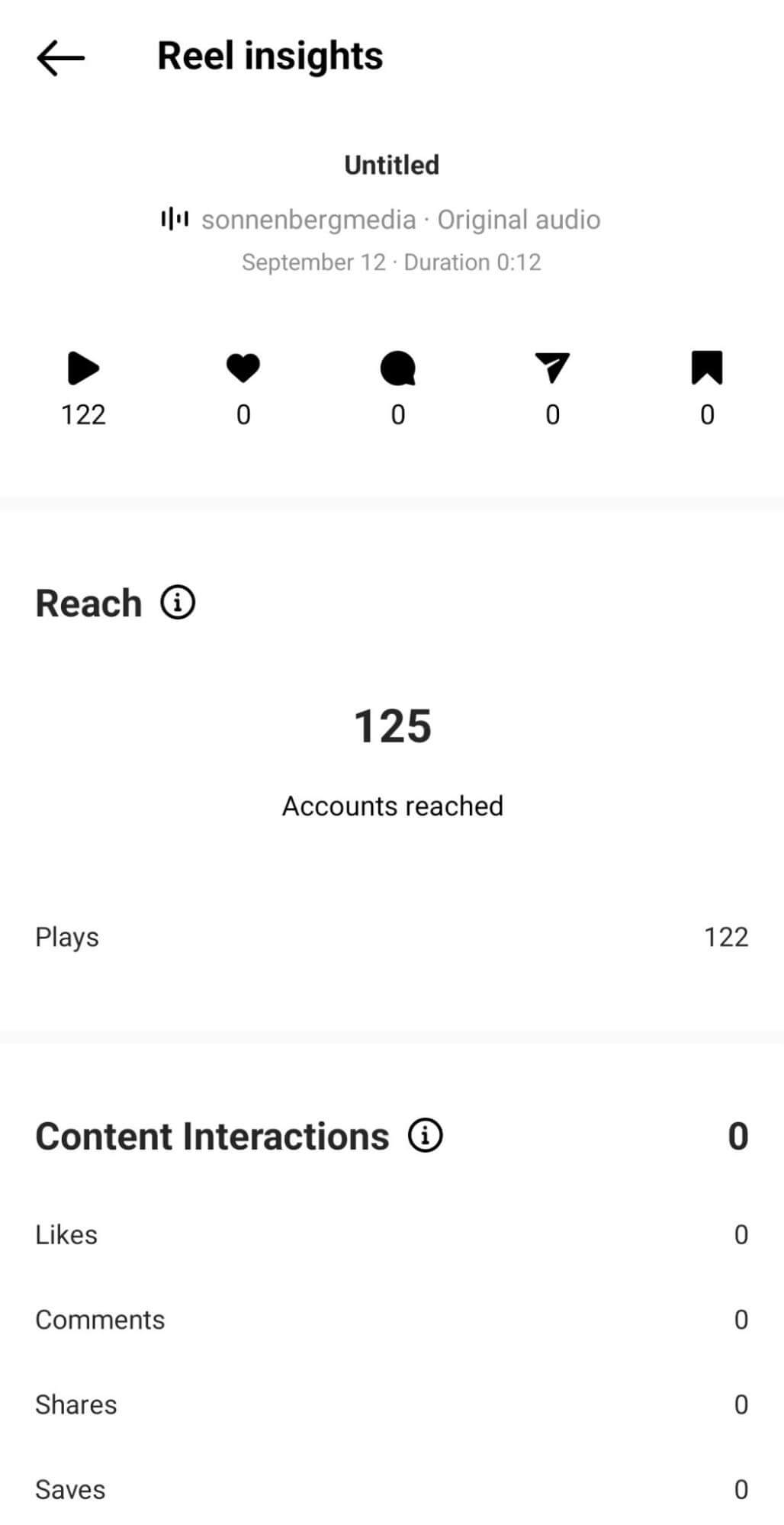This image appears to be a detailed screenshot from a media analytics platform called "Real Insights" (spelled R-E-E-L Insights). At the top left corner, there is a black arrow icon pointing to the left next to the platform's name. The page is titled "Untitled." 

Directly below the title, there's a waveform graphic indicative of audio analysis, labeled "Sonnen Burra Media Original Audio," accompanied by a date and duration timestamp. 

Further down, the interface displays various interactive buttons—play, heart (likely for likes), comment, share, and bookmark. 

The section beneath these buttons is labeled "Reach," with an information icon providing extra details. The metrics show "125 Accounts Reached" and "122 Plays."

Below this, there's a section titled "Content Interactions," again with an information icon. It lists various interaction metrics including Likes, Comments, Shares, and Saves, each showing a count of zero.